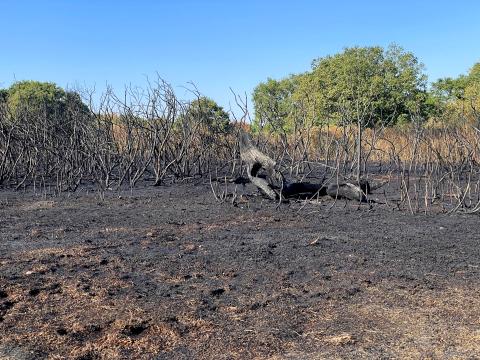The image depicts a small square outdoor scene set in a dry, semi-arid field. At the top of the picture, the sky is a clear, uninterrupted blue, devoid of clouds. Beneath the sky, there are taller, lush green trees lining the background, including a fairly large rounded tree to the left and some deciduous trees to the right. The middle ground shows evidence of a burnt or extremely dry area, with bare, leafless branches and bushes sticking up from the ground, making the area appear charred. The ground itself shows a contrast from dark brown and black—resembling ash—to lighter brown tones toward the bottom of the image. Among the barren branches in the center of the picture, there appears to be an unidentifiable brown object, possibly the remains of a structure, or a carcass showing hues of white, gray, and black. The foreground contains patches of dry grasses, dirt, chopped up grass, and twigs, accentuating the desolate and arid nature of this landscape.